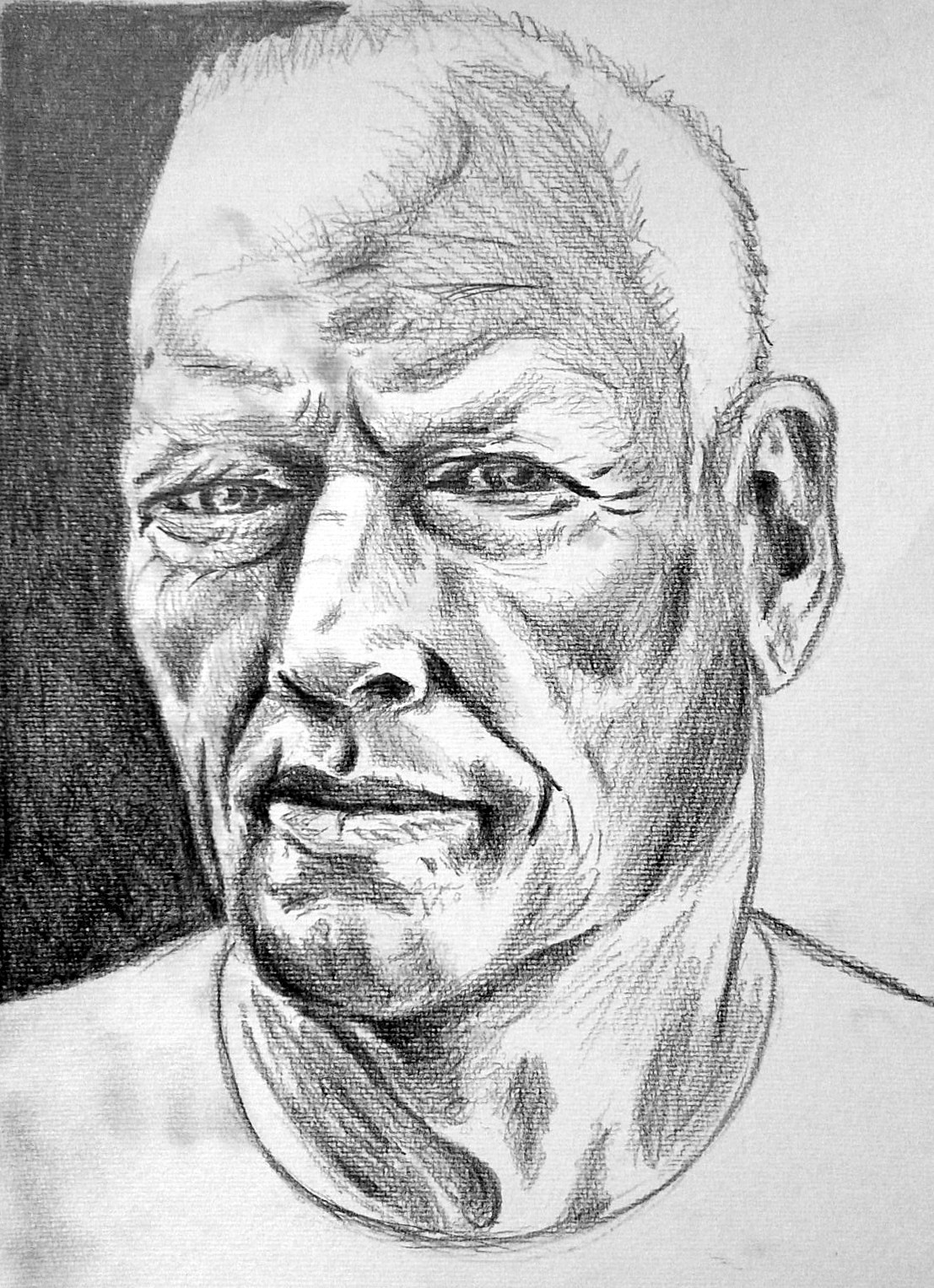This charcoal drawing portrays a Caucasian man who appears to be around 70 years old. His deeply etched facial features reveal a wrinkled brow and pronounced lines around his mouth. He has light-colored eyes that gaze intently straight ahead, enhanced by the stark contrast of his white or very light blonde hair. His hair is partially swept over his forehead, with a noticeable receding hairline on the upper right side. The left side of his head is heavily shaded in black, creating a dramatic contrast with the unshaded right side. The shadows cast on his neck further emphasize the depth and texture of the drawing. He wears a simple T-shirt, lacking a prominent collar, which keeps the focus on his expressive face. The man's serious expression adds to the overall intensity and realism of the artwork.